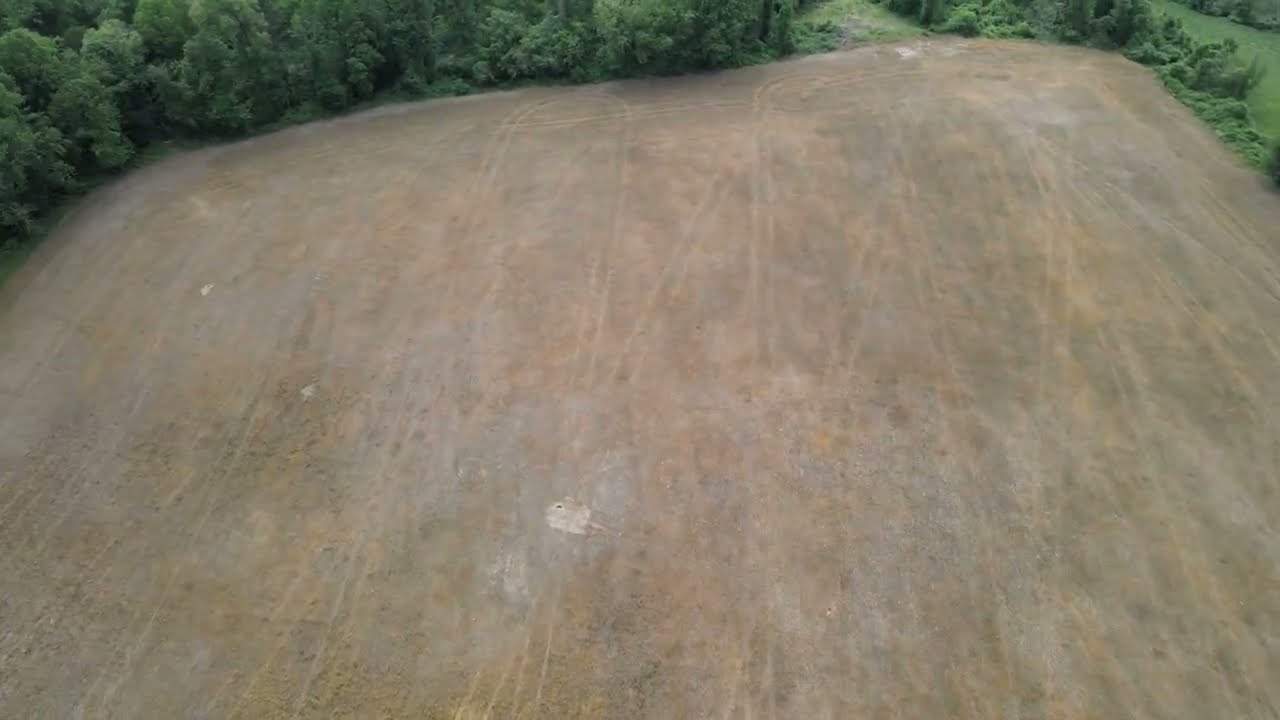This is an aerial photo of a large field with light brown soil, occupying the majority of the image. The field appears either recently harvested or newly planted, as it shows extensive vehicle tracks in both diagonal and straight patterns crisscrossing its surface. Scattered throughout are patches of gravel and dirt, contributing to the uneven texture of the terrain. The field itself has a rectangular shape, though its borders are not perfectly square, with curved corners giving way to straight edges.

Surrounding this expansive dirt area is a thick tree line, creating a vivid contrast with its lush foliage. The trees exhibit a range of greens, from dark, shadowy hues to brighter, lively shades, interspersed with grassy patches. Notably, the bottom left and right of the image lack tree coverage, where the field extends beyond the frame. In the top right corner, the woodland appears denser, with a diverse canopy. Additionally, there seems to be a pathway cutting through the wooded area on the center-right, hinting at some human activity or access route.